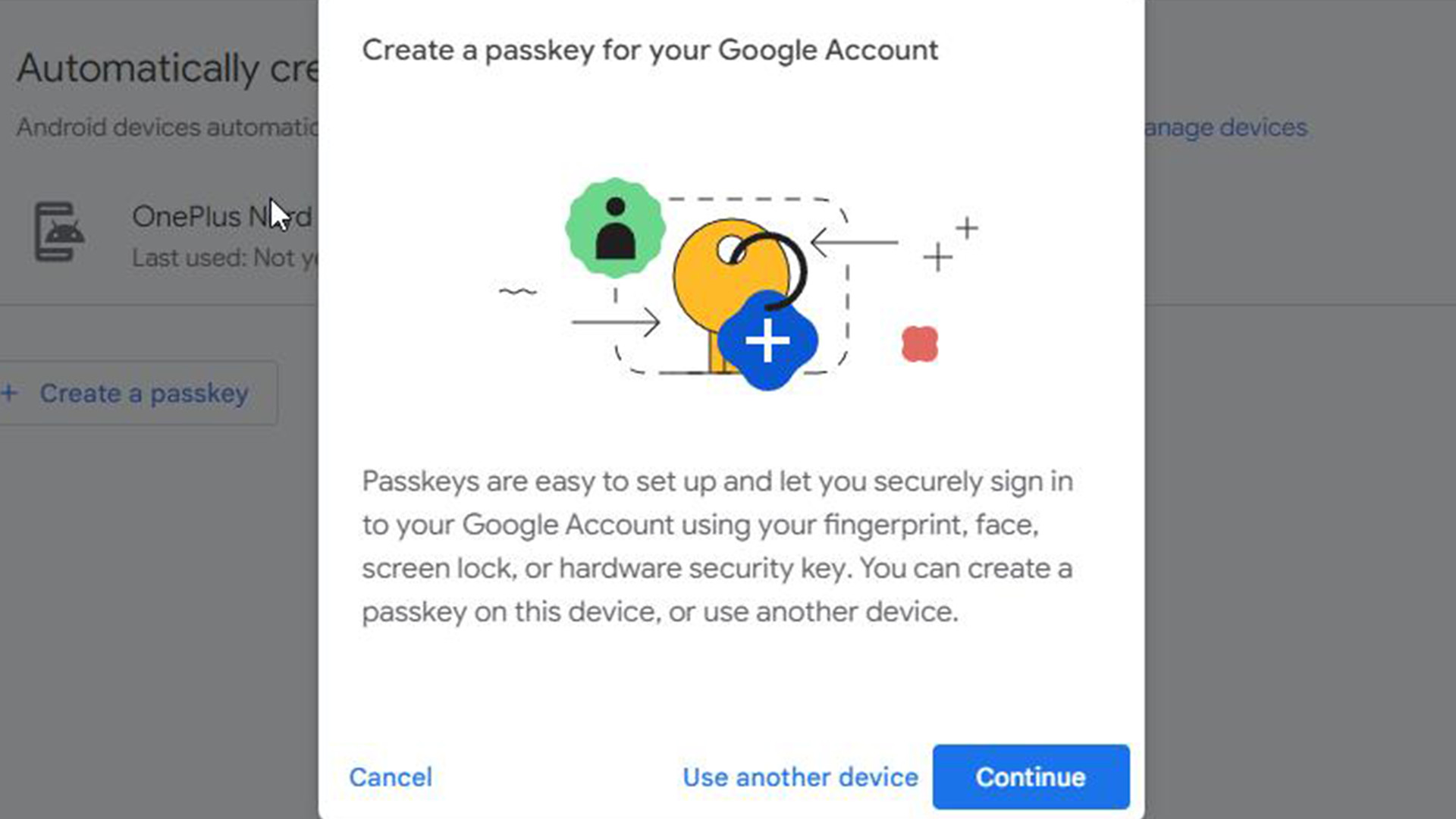The image depicts a cell phone screen with an overlay interface for creating a passkey for a Google account. The background is a gray, landscape-oriented rectangle displaying partially visible text and buttons. Overlaying this is a white, portrait-oriented rectangle that appears to have been generated after a user clicked something on the gray screen.

At the top of the white overlay, in dark letters, it reads: "Create a passkey for your Google account." Below this title is an illustrative diagram comprised of several components:
  - A yellow key icon in the center
  - A blue diamond with a white plus sign below the key
  - A green circle with a black person icon to the key's upper left
  - Dotted lines, rectangles, arrows, and additional plus signs connecting these elements, suggesting a flowchart or process diagram

Beneath the diagram is explanatory text stating: "Passkeys are easy to set up and let you securely sign in to your Google account using your fingerprint, face, screen lock, or hardware security key. You can create a passkey on this device or use another device."

At the bottom of the white rectangle, the options are provided:
  - "Cancel" in blue letters at the bottom left
  - "Use another device" in blue letters farther to the right
  - A blue button at the bottom right labeled "Continue" in white letters

The gray background screen includes partially visible text at the top left:
  - "automatically CRE"
  - "Android devices automatically"
  - "one plus last used"
  - A blue button with "create a passkey" as a clickable option

The information on the background screen is truncated and partially obscured by the white overlay.